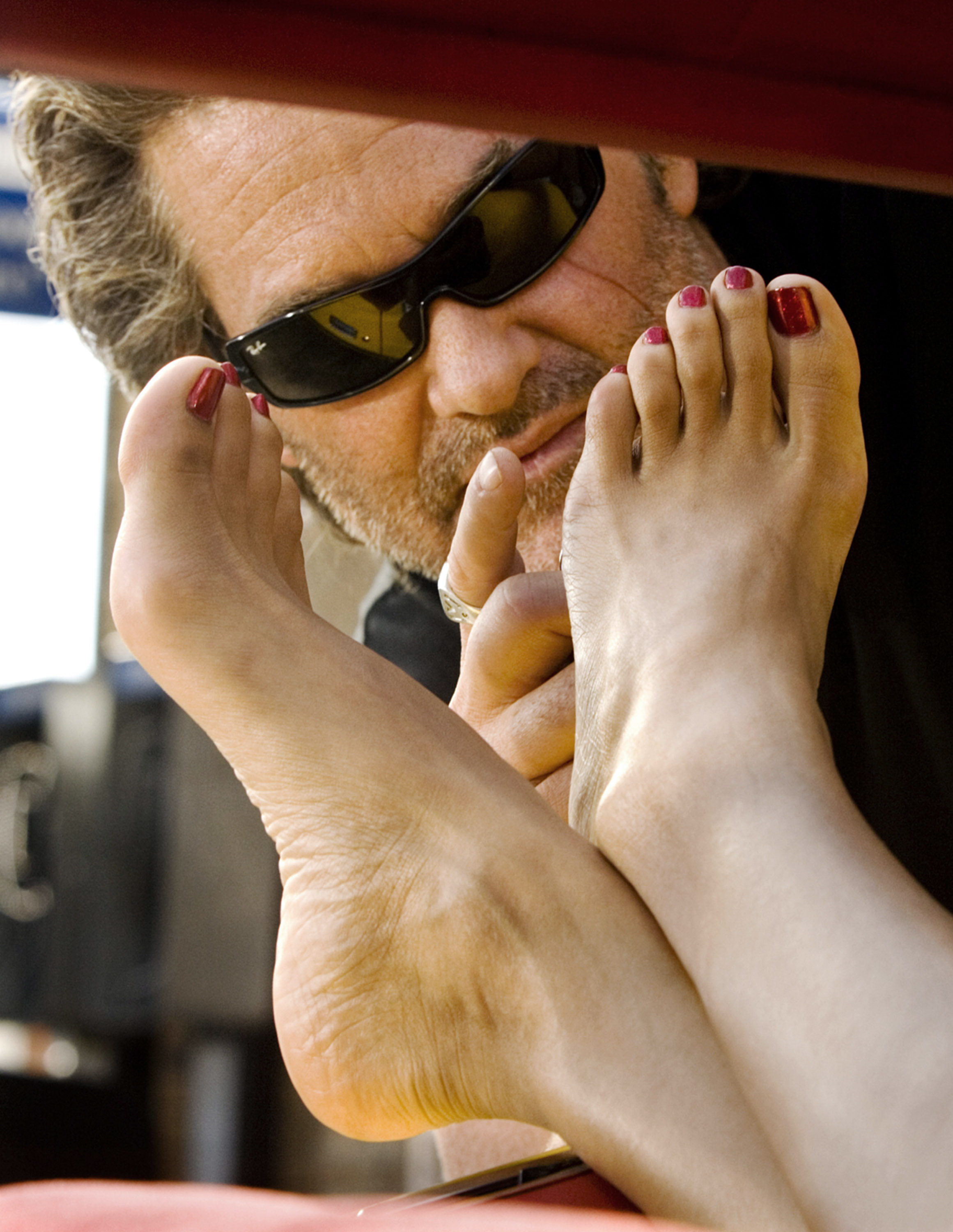The image showcases a scene likely from a film or TV show, where two white feet with red-painted toenails are prominently displayed, crisscrossed, and resting out of a car window, appearing through the window frame. One foot points left while the other faces a man in the background. This man, with gray hair and a beard, sports dark black sunglasses and has a scar down his left cheek. He reaches out to touch the bottom of one foot, with his index finger slightly lifted, adorned with a ring. He is framed against an out-of-focus background that includes some lighting, his head tilted at an angle. His sunglasses reflect what appears to be the scene around them.